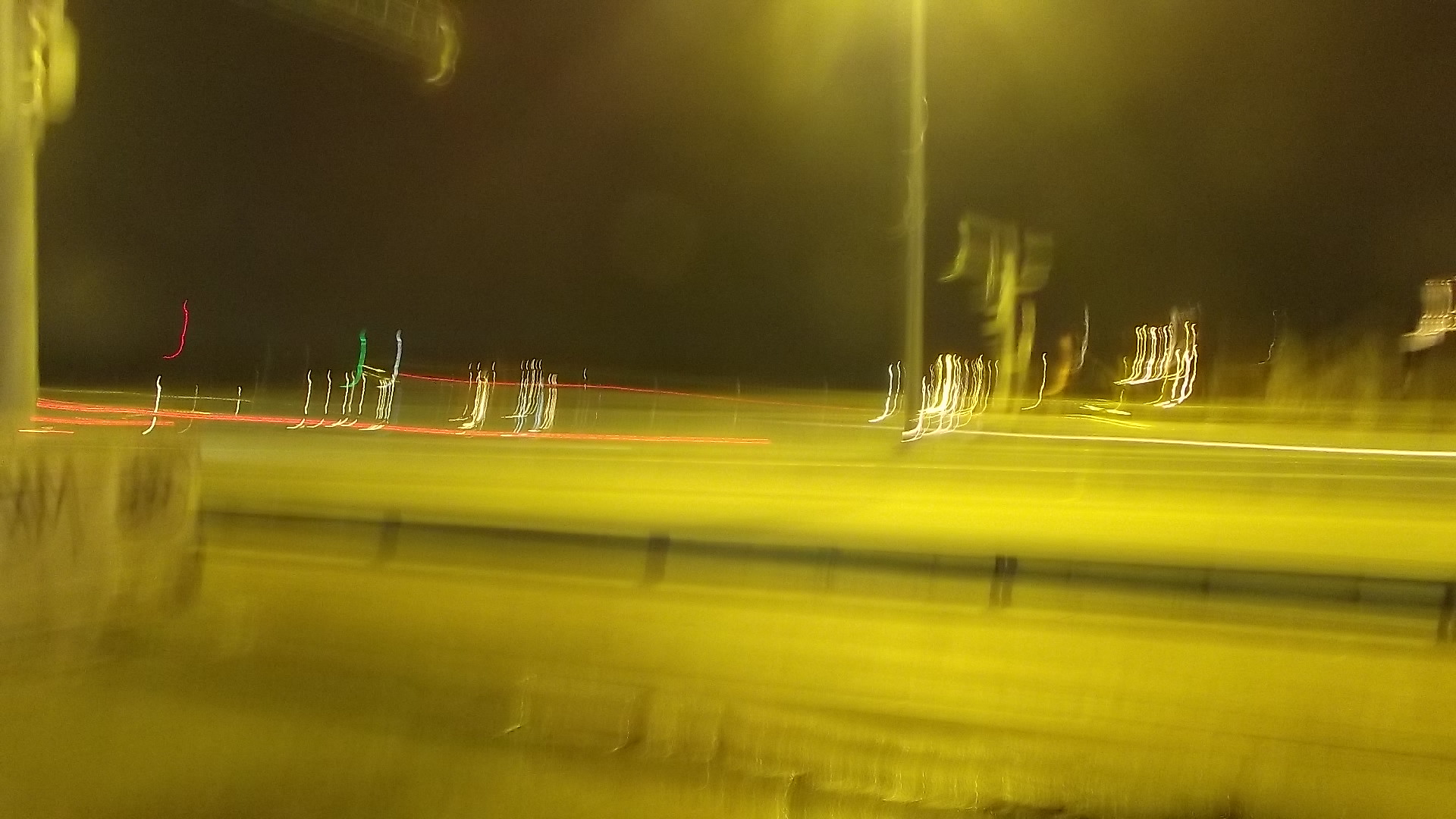This photograph, taken at night, captures the dynamic essence of a bustling highway, though it's rendered in a striking blur, suggesting rapid camera movement or a time-lapse capture. The sky, pitch-black, forms a striking backdrop to the scene below. Ghostly remnants of headlights and taillights trace vibrant streaks across the image in hues of white, red, and a singular green—each one a testament to the brief passage of unseen cars. Streetlights cast an orange glow that permeates the image, subtly illuminating the details within the chaotic blur. Light poles and guardrails frame the forefront and background, standing as silent sentinels to the constant motion. Weeds along the roadside add a touch of nature to this otherwise frenetic depiction of modern transportation.